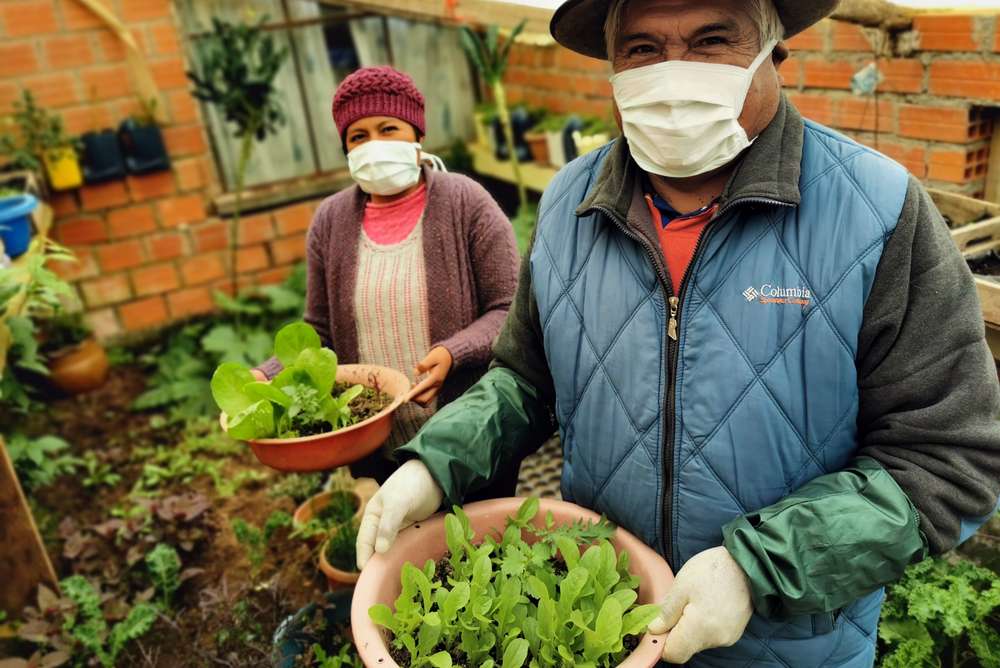The image depicts a man and a woman standing outdoors against a background of orange brick walls and a curtained window framed with brown panes. In front of the building, there are garden plots filled with green plants. Both individuals, likely Hispanic, are wearing white face masks. The woman, positioned on the left, is wearing a red beanie, a dark red cardigan over a white and red striped shirt, and another bright red shirt beneath. She is holding a bowl with soil and a plant that has larger green leaves. The man, on the right, is wearing a hat and a blue Columbia jacket with black sleeves and a green edge. He is also holding a similar bowl, but the plant inside has smaller leaves. Both individuals are looking up at the camera, and the well-lit setting suggests the image was taken during the daytime.